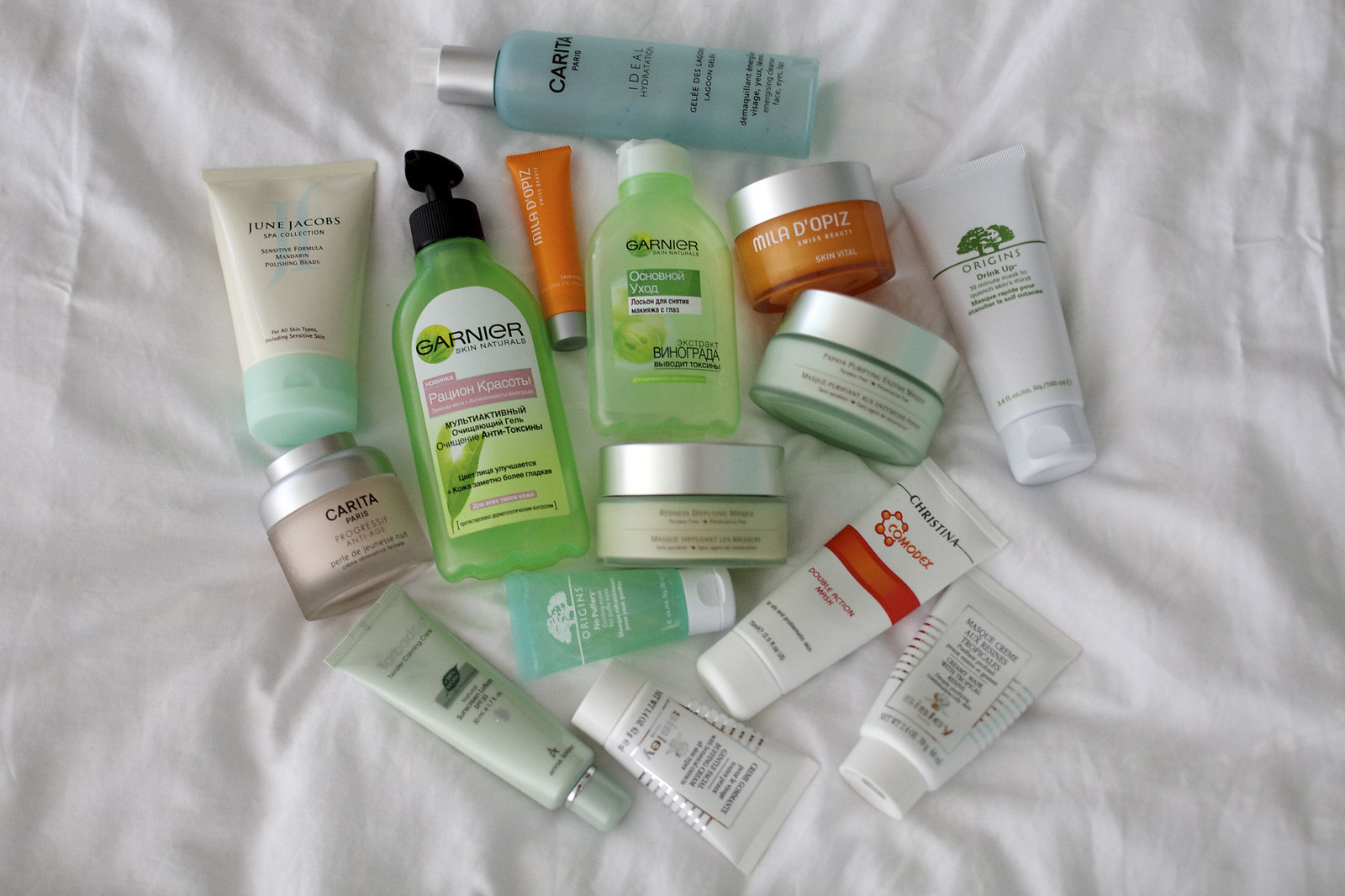This photograph showcases a diverse assortment of personal care and hygiene products meticulously arranged on a white fabric background, resembling a bed sheet. The collection features an array of bottles and tubes in different shapes and sizes. Prominently, a cylindrical bottle stands out at the top, distinguished by its blue hue and capped with a tall, silver top.

Several bottles exhibit rectangular shapes with gracefully curved shoulders. Among them, one notable bottle features a black screw cap paired with a triangular pump dispenser. Scattered around the central items, numerous white tubes face random directions, collectively forming a loose circular arrangement.

Some products from the Garnier line are evident, housed in clear plastic bottles with vibrant green contents. An Origins product features a clear plastic tube with a white cap, revealing a blue-green substance within. Additionally, a long, white, opaque tube from Origins is positioned on the right side, adorned with a green tree logo at the top. This careful presentation invites a closer look at the variety and specificity of the personal care items displayed.